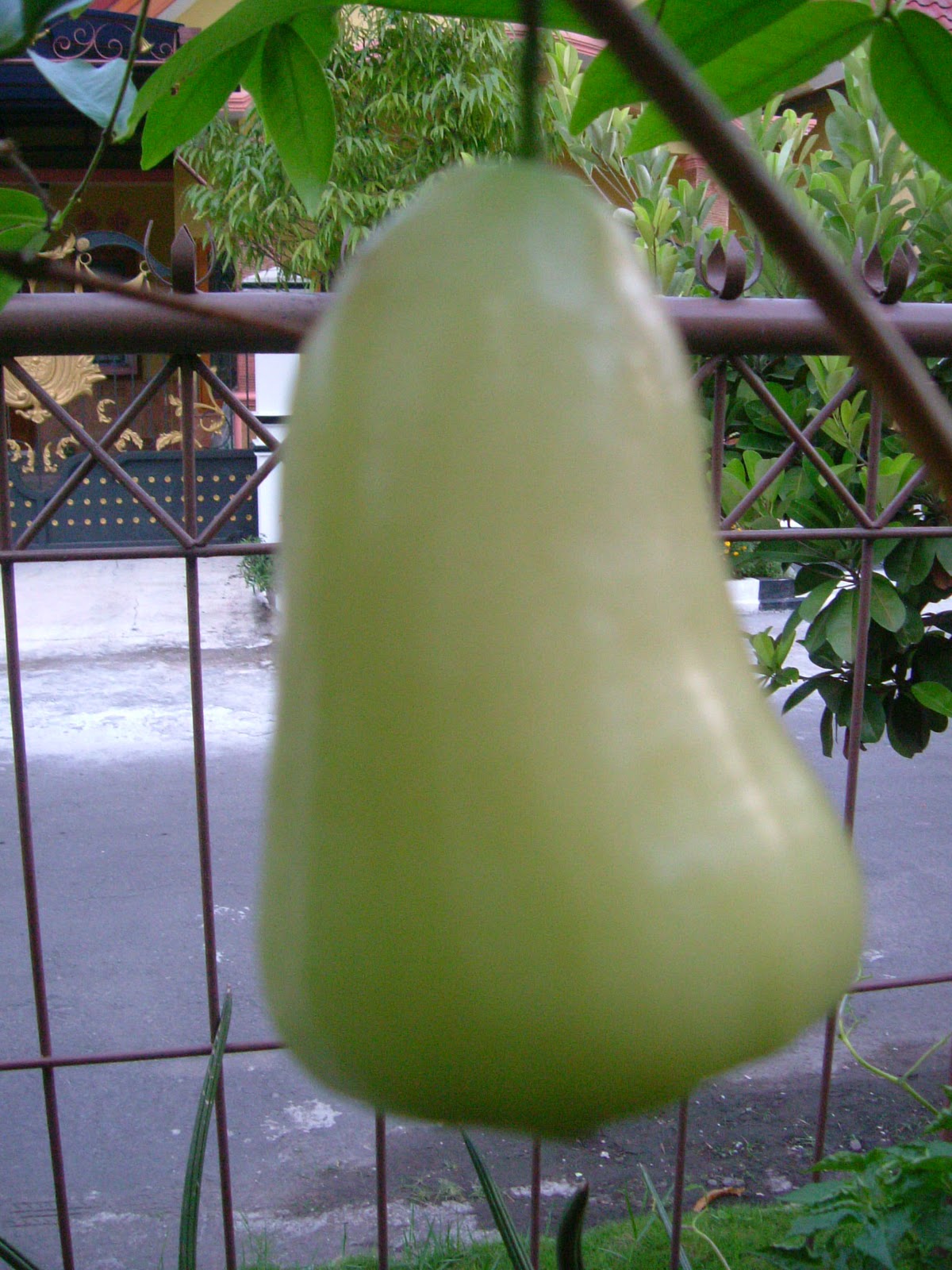This photograph captures a detailed scene centered around a large, light green pear-like fruit hanging from a tree or plant. The fruit, appearing larger than average and probably ripe, is slightly out of focus, emphasizing the background details. Surrounding the pear, you can see the brown branches of the tree and green grass below it. Behind the fruit stands a sturdy, metal, bronze-colored fence or trellis. In the background, there is a white building, possibly a temple, partially obscured by the structure. The area is filled with greenery, including trees, bushes, and additional plants hanging down. The ground beneath appears to be a mix of light gray cement and a white sidewalk. This close-up garden shot provides an intimate look at the natural setting around the fruit.